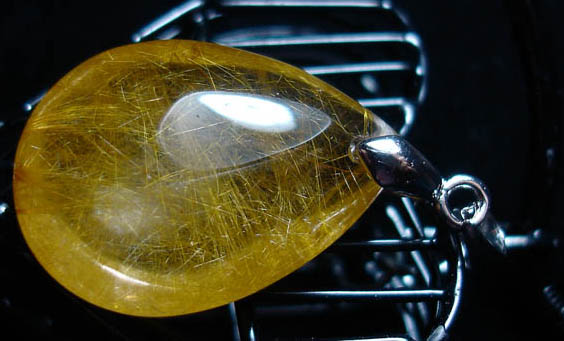The photograph features a very close-up image of a pendant, likely part of a necklace, with a teardrop shape. The pendant appears to be yellowish in color, with an amber-like, muted translucency that hints at it being a gemstone or a rock. It is securely affixed to the necklace with a metallic clasp, though no chain is visible as the image cuts off before that point. The pendant rests upon a heart-shaped metal piece, adding to its decorative appeal. The entire composition is set against a stark black background, enhancing the elegance of the amber-yellow color and the metallic attachments. The image focuses exclusively on the pendant and its immediate surroundings, capturing intricate details and textures, making it a striking and somewhat abstract piece of art.